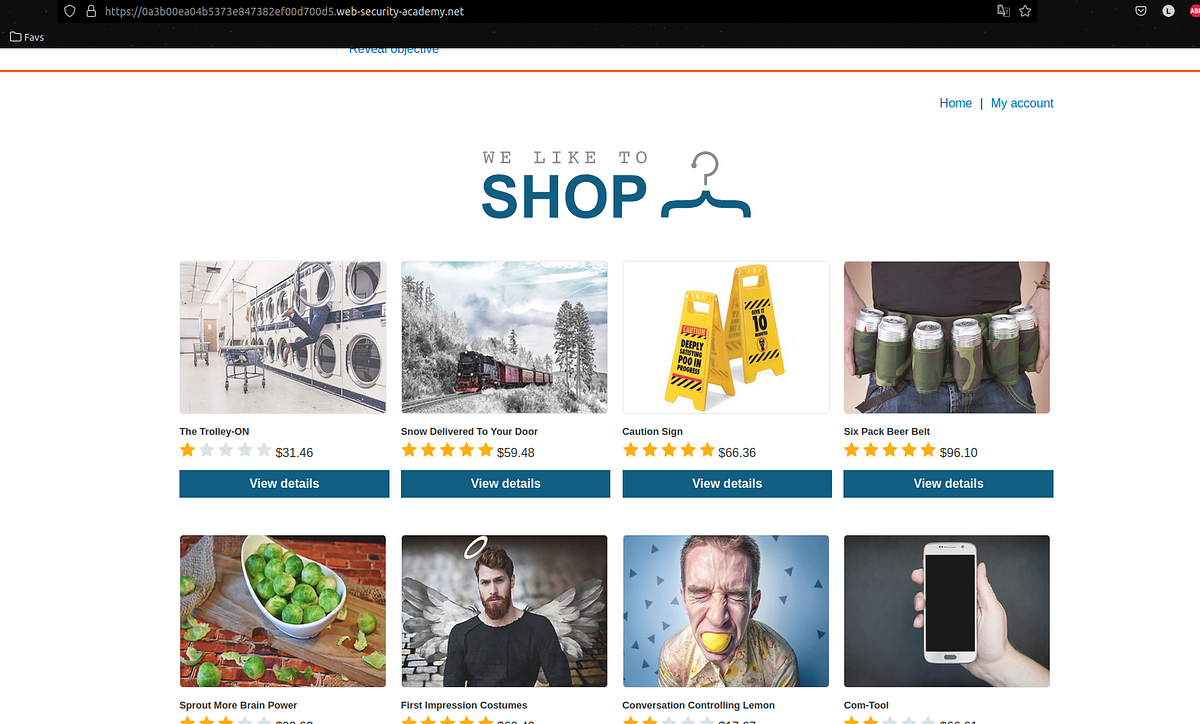This image is a detailed screenshot of an online shopping website, showcasing a user-friendly interface designed to facilitate easy browsing and purchasing of products. At the top center of the screenshot, there is a logo featuring text that reads "We'd Like to Shop," accompanied by a coat hanger icon, indicating the site's focus on various shopping items.

The central area of the webpage prominently displays eight product images arranged neatly in two rows of four. Each product is accompanied by a brief description and relevant details, such as:
- "Snow Delivered to Your Door"
- "Six-Pack Beer Belt"
- "Cam Tool"
- "Caution Sign" (illustrated with a picture of two yellow caution signs resembling those used to indicate wet floors).

Each product listing includes additional information such as price, user ratings out of five stars, and a large blue button labeled "View Details." This button is intended to lead users to more comprehensive information about the product, including additional images, detailed descriptions, and purchasing options.

In the top right corner of the screen, there are two blue text links labeled "Home" and "My Account," allowing users to return to the homepage or manage their account details. The top of the screenshot features a large black bar, which is the web browser's address bar currently showing the URL of the shopping website. Overall, the screenshot captures the essential elements of the online shopping experience offered by this website.